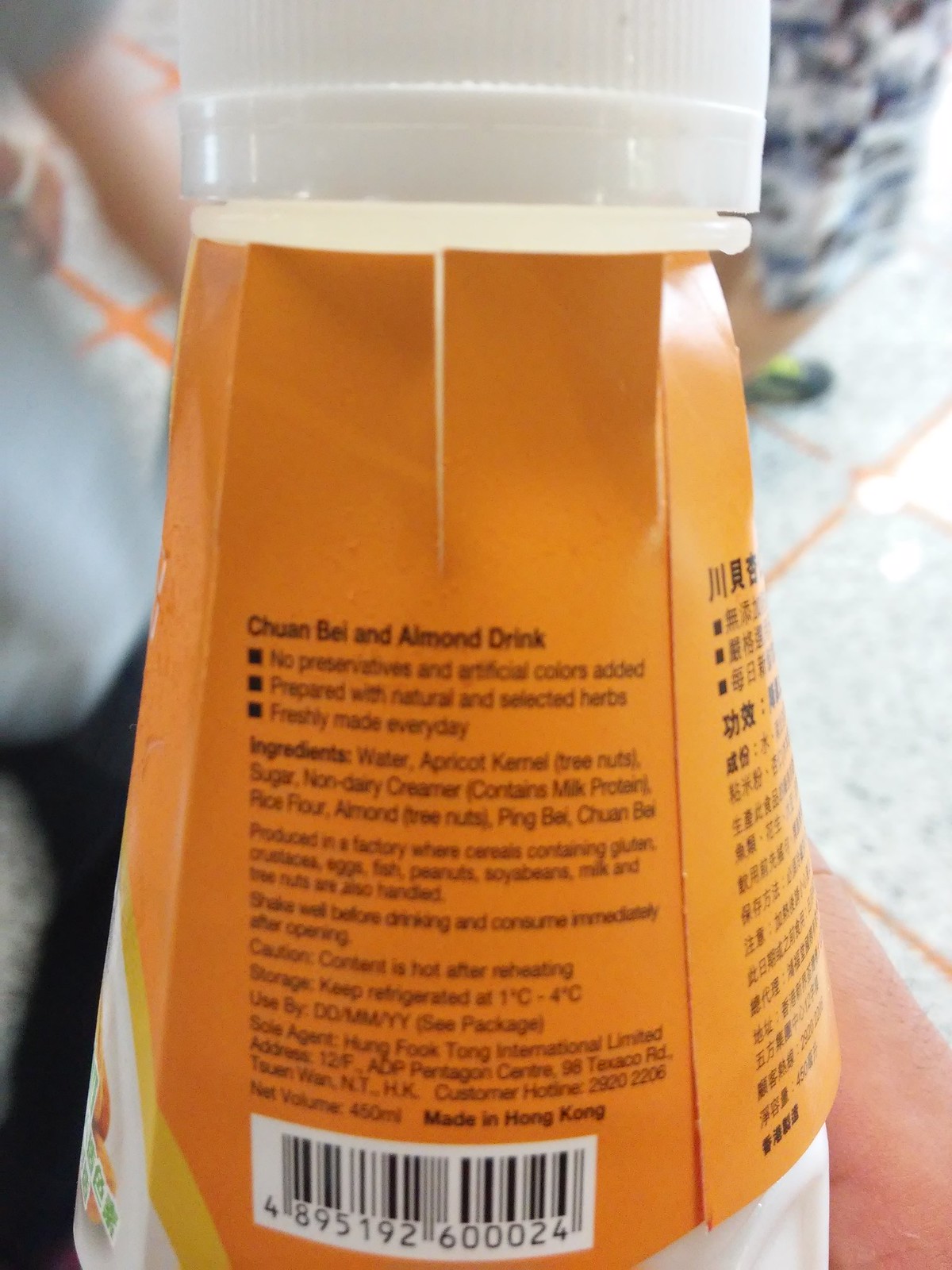The image features a vertically-oriented, slightly conical, cardboard bottle of a food product, filling the frame from top to bottom. The bottle's top and bottom edges are slightly cut off, leaving ample space on both the right and left sides of the image. The body of the bottle narrows slightly as it ascends, with the top circle's diameter approximately 70% of the bottom's diameter. The container appears to be hexagonal or octagonal due to visible ridges, giving it a polygonal shape.

The back label of the bottle is the focal point, prominently featuring text in both English and Chinese. The label is mainly a light orangish-brown. Near the middle of the label, the text "Chuan Bai and Almond Drink" is displayed prominently. Below this, there are three block bullet points, the first of which states "no preservatives and artificial colors added." An ingredients list follows, starting with "Ingredients: Water, apricot kernel," in bold font. Additional lines list other ingredients and note that the product is manufactured in a facility that processes gluten-containing food, although this text becomes progressively smaller.

Further down, there's a caution regarding the product being hot after reheating and storage instructions, "Keep refrigerated at 1°C - 4°C." The bottom right of the label states "Made in Hong Kong" in bold type, accompanied by a rectangular UPC symbol at the bottom.

The top of the bottle features a white plastic, ridged twist-off cap, visible though not fully captured in the image. The surrounding background reveals light gray flooring with dark orange checkerboard patterns.